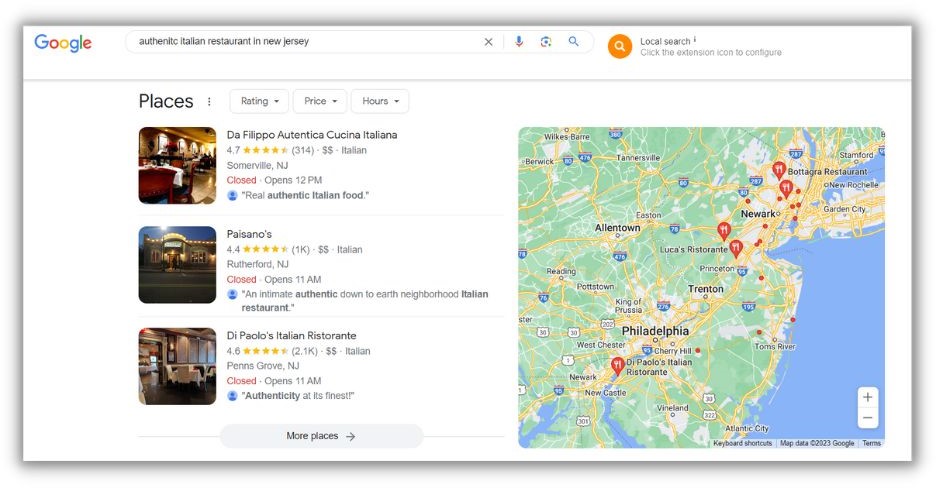The image displays a Google search result for "Authentic Italian Restaurant in New Jersey." On the left, the classic Google icon is prominently featured, while to its right, there is a search bar containing the query. Adjacent to the search bar, an orange magnifying glass labeled "Local Search" is clearly visible. Below the search area, a large, detailed map showcases key cities including Philadelphia, Newark, Trenton, and Allentown, essentially covering all of New Jersey with notable cities marked and the ocean on the right side.

On the left side of the map, there is a filter tab labeled "Places," which allows sorting by ratings, price, and hours of operation. Under this tab, there are results for three Italian restaurants: Paziano's, La Filippo Ottica Cucina Italiana, and Di Pablo's Italian Ristorante. Each restaurant entry provides detailed information including ratings, pricing, cuisine type, and operating hours. Additionally, a "More Places" tab is located in the middle-right section of the image, offering further search options for additional restaurants.